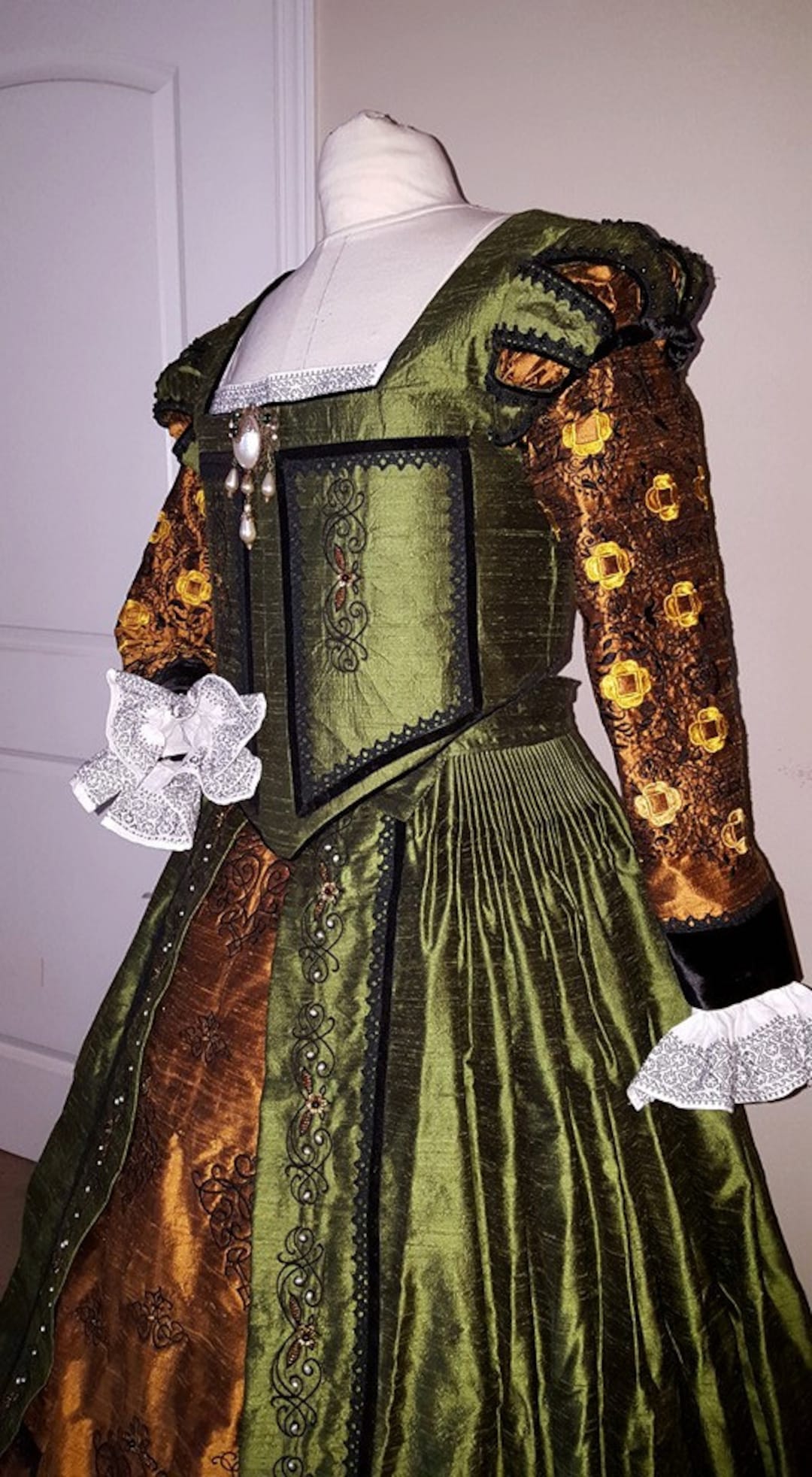The image depicts an intricately designed, headless and armless white mannequin adorned in a lavish, Renaissance or Elizabethan-era dress, suitable for a setting reminiscent of a Game of Thrones-type TV show. The dress, primarily a rich olive green, features a low-cut neckline that allows a glimpse of cleavage and is accented with a black detail on the belly area. The bodice, resembling a corset, is fitted and fastened with white fasteners, while the shoulders are designed to be poofy.

On the mannequin's arms, the dress covers a shirt with gold sleeves adorned with delicate yellow floral patterns and finished with billowy white ruffles at the cuffs. This shirt gives the sleeves a coppery color, adding an additional layer of richness to the attire. The floor-length skirt of the dress is flowy with green panels on either side, contrasted by a central orange or copper strip, creating a striking visual balance.

The setting appears to be indoors with a cream-colored wall to the right and a semi-decorative white wooden door to the left, emphasizing the historic and luxurious nature of the garment. There is also a piece of jewelry adorning the chest area of the dress, further asserting the opulence and period style of the outfit.